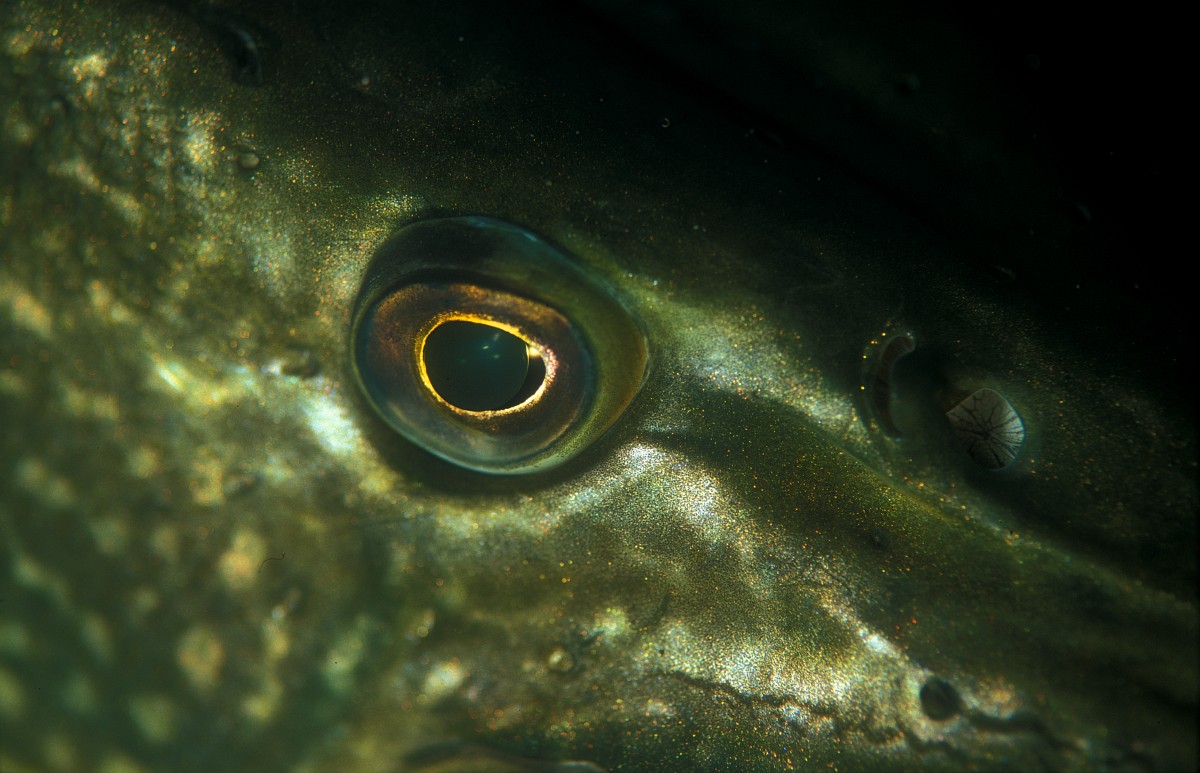This photograph features a striking close-up of a sea creature's eye, possibly belonging to a crocodile, alligator, or a large fish. The eye is prominently centered, showcasing its complex color pattern. The outermost part of the eye consists of a textured green circle, mottled with shades of dark green, light green, and gray-green. Encircling the dark centered pupil is a wide band of golden-gray, followed by a thinner, brighter yellow or light gray band. The skin surrounding the eye is primarily army green with a shiny luster, accentuated by gold specks and tinges of white. Set against a jet-black background, the image suggests an underwater environment, possibly deep in the ocean where details of other creatures remain obscured by darkness.